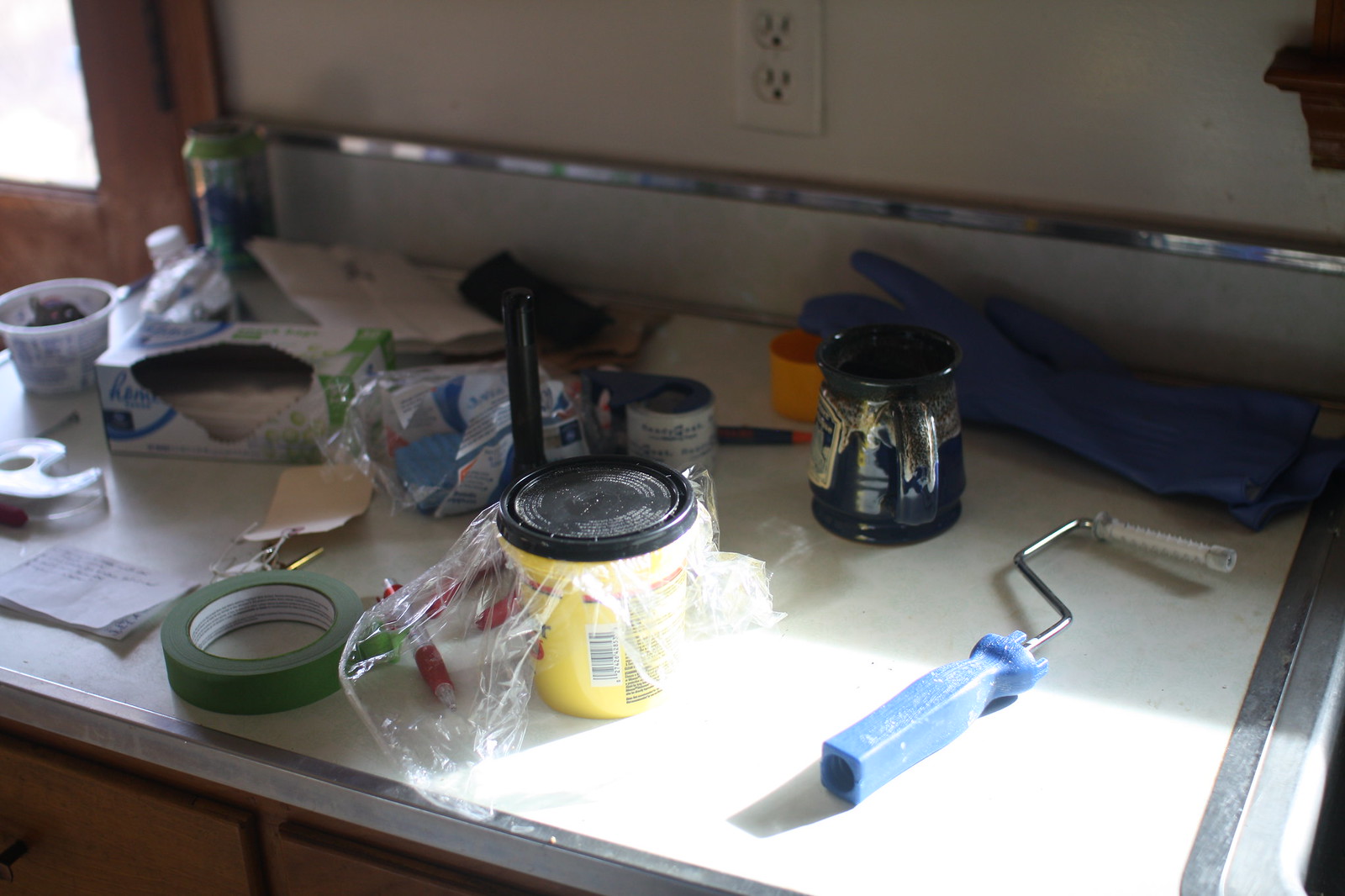This photograph captures a nostalgic kitchen, reminiscent of the 1950s to 1970s, featuring aged wooden cabinets and a stainless steel bound laminate countertop. Against a pristine white wall, an old-fashioned electric socket and a window framed in matching wood trim complete the charmingly vintage scene. Spread across the countertop is an array of tools and supplies, signaling an imminent home improvement project. 

A pair of blue rubber work gloves lies casually next to a coffee mug, an essential companion for any hands-on task. Painter's tape, plastic bags, sponges, and Scotch tape are scattered around, alongside a list and pens, hinting at a well-organized plan. A collection of trim brushes rests nearby, along with several containers filled with various tools and small items. Packing tape and a paint roller handle without its cover indicate preparations for painting. 

Towards the front, an opened container of putty or wood filler, sealed with saran wrap and capped to prevent drying, suggests some patchwork is already in progress. Additional items such as paper, containers, and the top of a spray paint can further emphasize the readiness for renovation. This glimpse into the past and the ensuing transformation encapsulates a moment of practical nostalgia and anticipation.